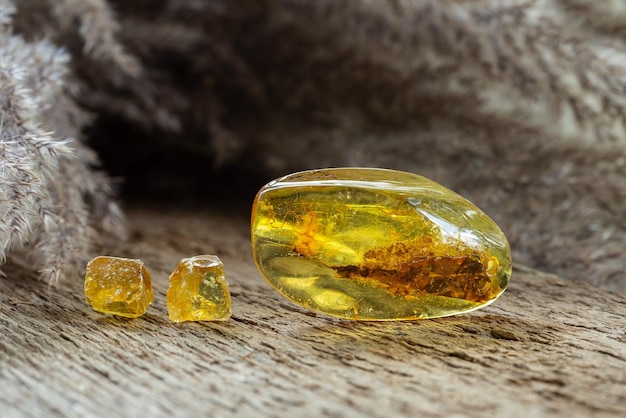The image features a close-up of three rocks or gemstones set against a light, slightly textured background. Slightly right of center, there is a prominent, large, smooth oval stone with a yellow, goldish hue, and varying shades of brown that widen towards the bottom right. This stone is semi-transparent and has an oblong shape. To the left of this larger stone are two smaller, roughly angular, cube-like stones of the same yellowish-amber color. They appear jagged but exhibit some smooth surfaces. The stones rest on what appears to be a wooden surface extending from the bottom right of the image towards the upper left. In the out-of-focus background, one can see white and dark-colored elements, possibly branches or plants, contributing to a somewhat fuzzy backdrop. Towards the top left, there are hints of wispy, plant-like structures in whitish shades.